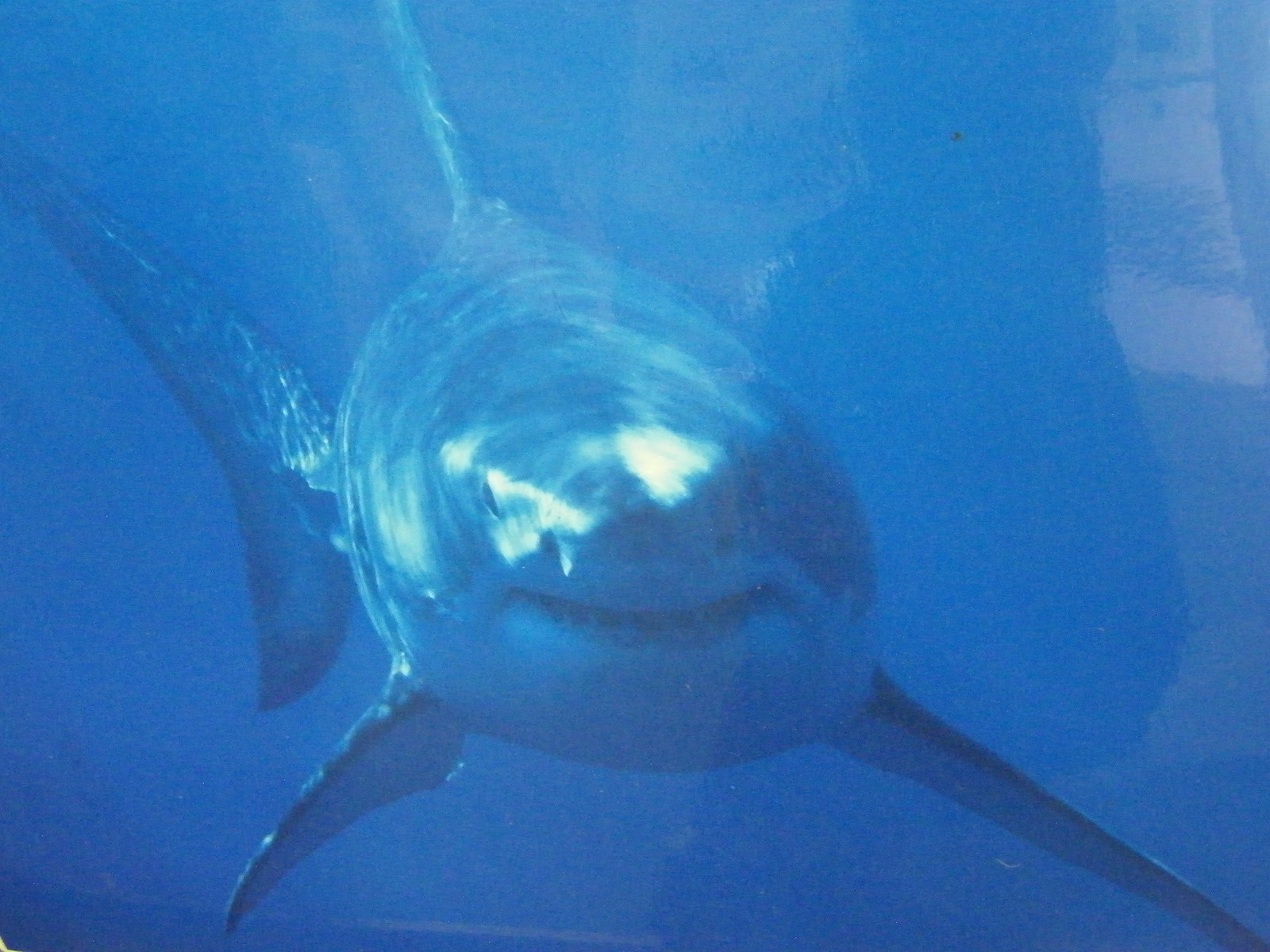This detailed image captures a large great white shark underwater, swimming directly towards the viewer. The shark has a formidable, gray body with a white underside and features distinct, beady black eyes on the sides of its head. Its mouth is open, revealing a row of sharp teeth, giving the illusion of a menacing smile. The shark's long fins extend across the image, with its dorsal fin prominent on its back and its tail fin visible towards the left side.

The underwater environment is a deep, dark blue, and the illumination suggests sunlight filtering down from above. The photograph has a glossy, reflective sheen, possibly indicating it is a photo of a photo or a large display poster. There are noticeable light reflections, including one glaring off the shark's eye, adding to the glossy appearance. On the upper right and extending down the right edge of the image, there's a pronounced shadow, which could be either a reflection or the photographer's shadow.

Overall, the image conveys a sense of being face-to-face with the shark, accentuated by the underwater backdrop and the realistic textures and lighting, which create a vivid, almost immersive experience.